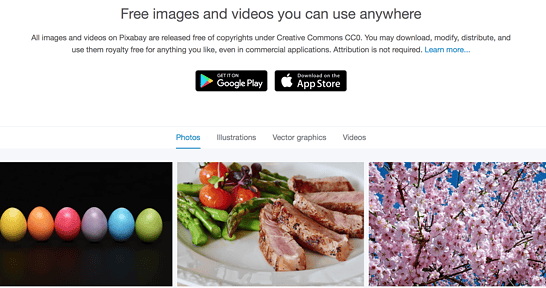Discover a world of royalty-free images and videos perfect for any use with Pixabay. All media files on Pixabay are released under Creative Commons CC0, meaning they are free of copyrights and can be downloaded, modified, distributed, and utilized without fee, even in commercial applications. No attribution is necessary. 

The app is available for download on Google Play, indicated by the Google Play logo, and the Apple App Store, signified by a white Apple logo. The platform offers a wide range of media including photos, illustrations, vector graphics, and videos.

In one highlighted image, a series of Easter eggs in vibrant colors—yellow, orange, red, gray, blue, and green—are aligned against a black background. Another image features a gourmet plate with sliced meat, asparagus, and tomatoes. Additionally, a beautiful photograph captures a cherry blossom tree in full bloom.

For more information and to download the app, visit www.pixabay.com.